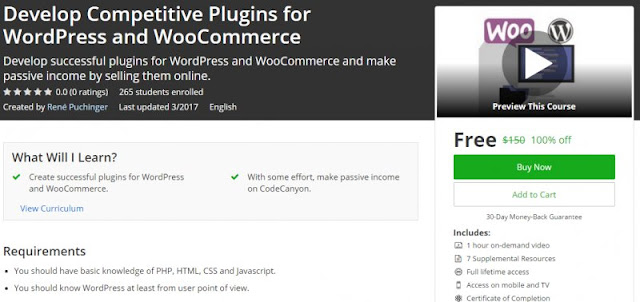The image features a prominent, dark brownish-black top bar that spans the entire width from left to right. On the left side of this bar, large white text reads, "Develop Competitive Plugins for WordPress and WooCommerce." Beneath this, in smaller font, it says, "Develop successful plugins for WordPress and WooCommerce and make passive income by selling them online." Below this description is a section showing a star rating, which currently has no ratings, and information stating that 265 students are enrolled. This course is created by Renee Puchinger and was last updated in March 2017. The language of instruction is English.

On the right side of the brownish-black bar, there is a preview video. Below this video, a title reads, "Preview this Course." A play button is centrally located within the video thumbnail. Additionally, the video is labeled "Free," with a crossed-out original price of $150, indicating the course is 100% off.